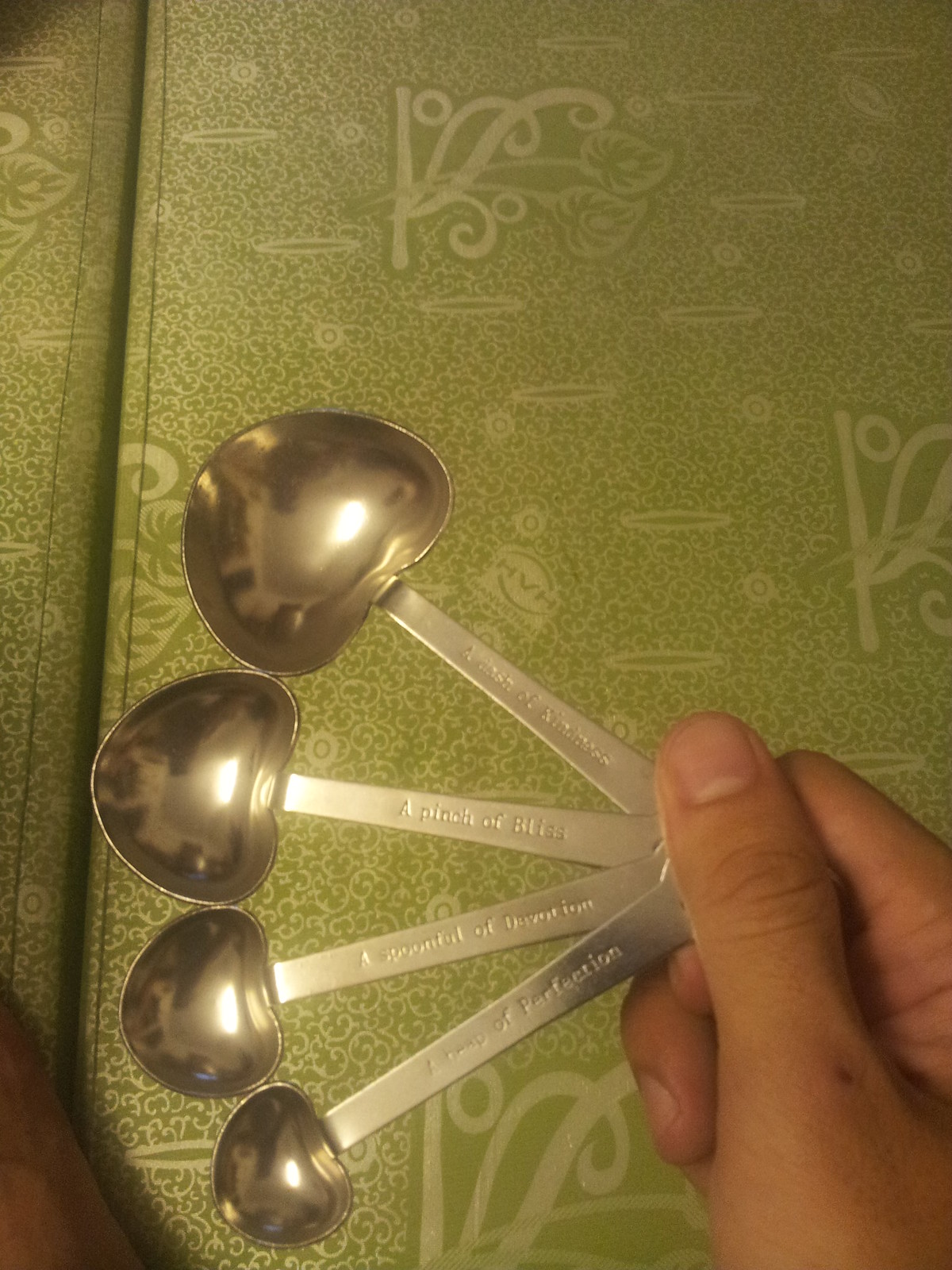This is a close-up photograph featuring a set of silver measuring spoons held by a light-skinned hand that enters the frame from the bottom right corner and extends towards the upper left. The fingers are wrapped around the spoons, with the thumb and visible fingernail prominently shown. The spoons are fanned out with the largest one on top and progressively smaller sizes below. The bowls of the spoons are slightly heart-shaped, wider at the part where they meet the handle and narrower at the tip, with a rounded design. Each spoon is inscribed with different whimsical measurements: "a pinch of bliss," "a dash of kindness," "a spoonful of devotion," and "a heap of perfection." The background is a mottled green surface, with swirling patterns and leaf images, possibly the cover of a book or a table draped in plastic. The spoons themselves are shiny and clean, reflecting light from their polished surfaces.